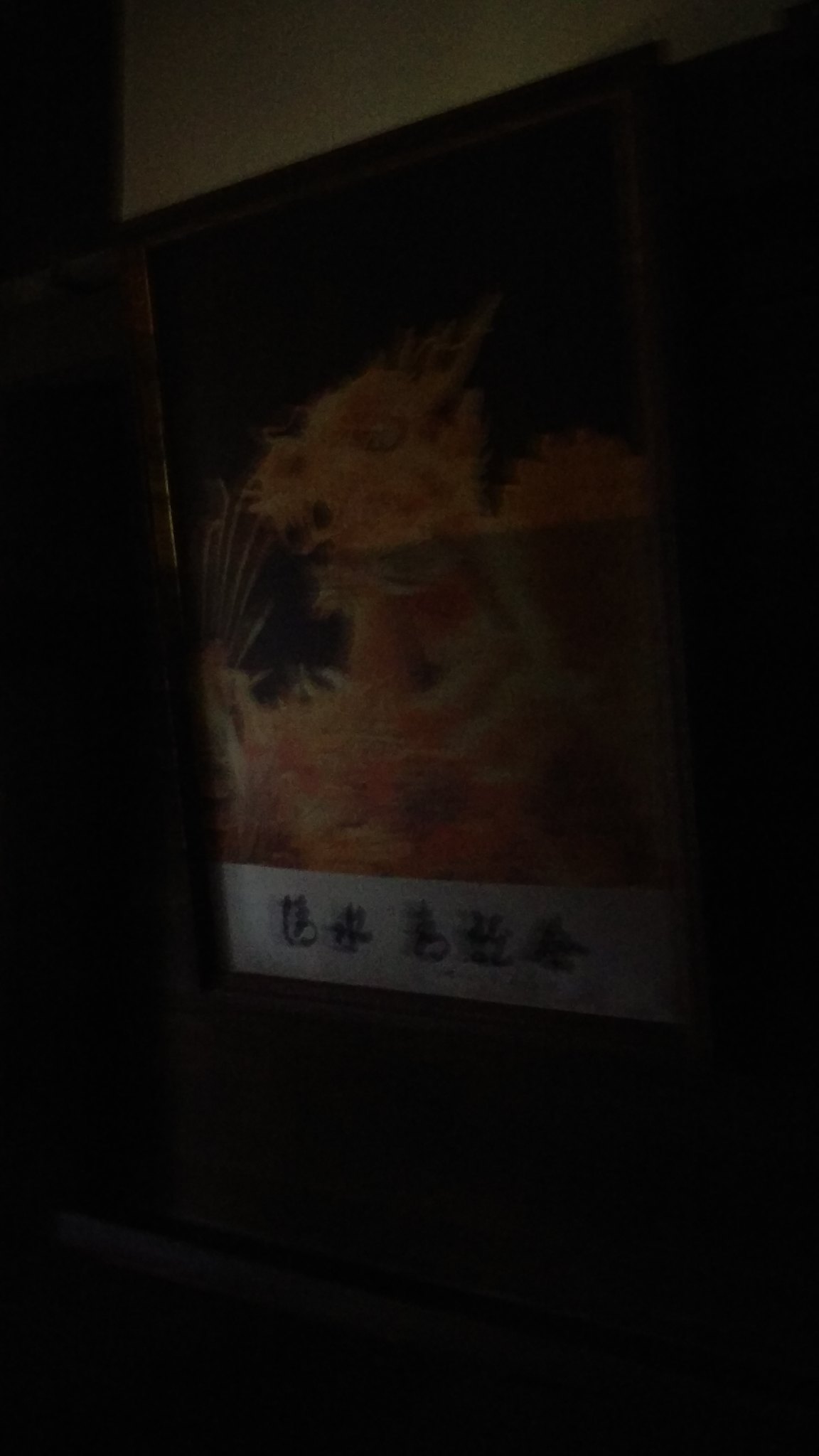This predominantly dark image features a framed poster or painting centered against a mostly black background. The wall at the top of the image is a light cream or gray color, transitioning to black on the outer edges and beneath the poster. The central image within the frame depicts the head of an animal, possibly a cat or dragon, characterized by round eyes, pointy ears, a snout-like nose, and an open mouth, rendered in orange and reddish hues with golden or sun-like outlines. Below this image, a white banner with black Asian-style writing is visible, although the exact characters are obscured by the darkness. The overall scene is dimly lit, contributing to the predominantly black appearance of the photograph.